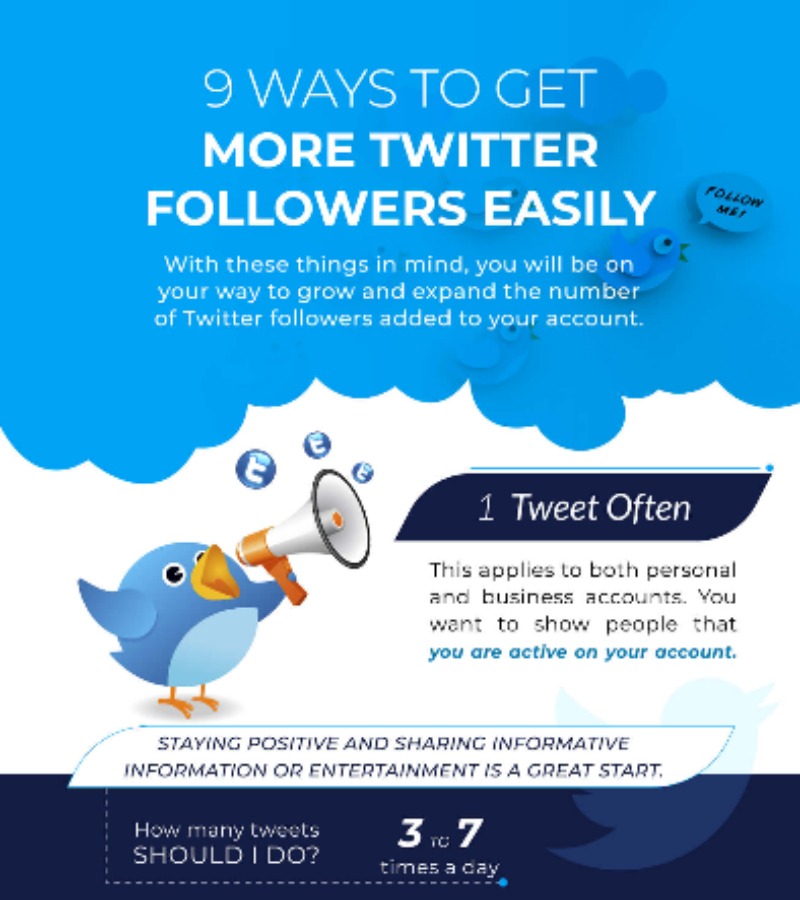The image features a vibrant and dynamic composition designed to provide tips on gaining more Twitter followers. 

At the top, a bright blue background sets the tone for the visual. On the right, two small animated birds are depicted, with one bird holding a speech bubble that reads, "Follow me." 

Accompanying text in white says, "Nine ways to get more Twitter followers easily." Beneath this, additional text explains, "With these things in mind, you will be on your way to grow and expand the number of Twitter followers added to your account."

Further down, the animated bird reappears with its orange beak open, this time holding an orange and white megaphone. Words emanate from the megaphone into a dark blue square, stating, "One: Tweet often."

Below this, text advises that this applies to both personal and business accounts, emphasizing that "you want to show people that you are active on your account," with "you are active" highlighted in blue.

Additionally, another box offers guidance: "Staying positive and sharing informative information or entertainment is a great start." 

At the bottom, a dark blue rectangle poses the question, "How many tweets should I do?" 

In bold white font, the answer "3-7" appears, followed by "times a day" underneath. The Twitter bird icon is positioned on the right side of this informative section, completing the instructional and engaging design.